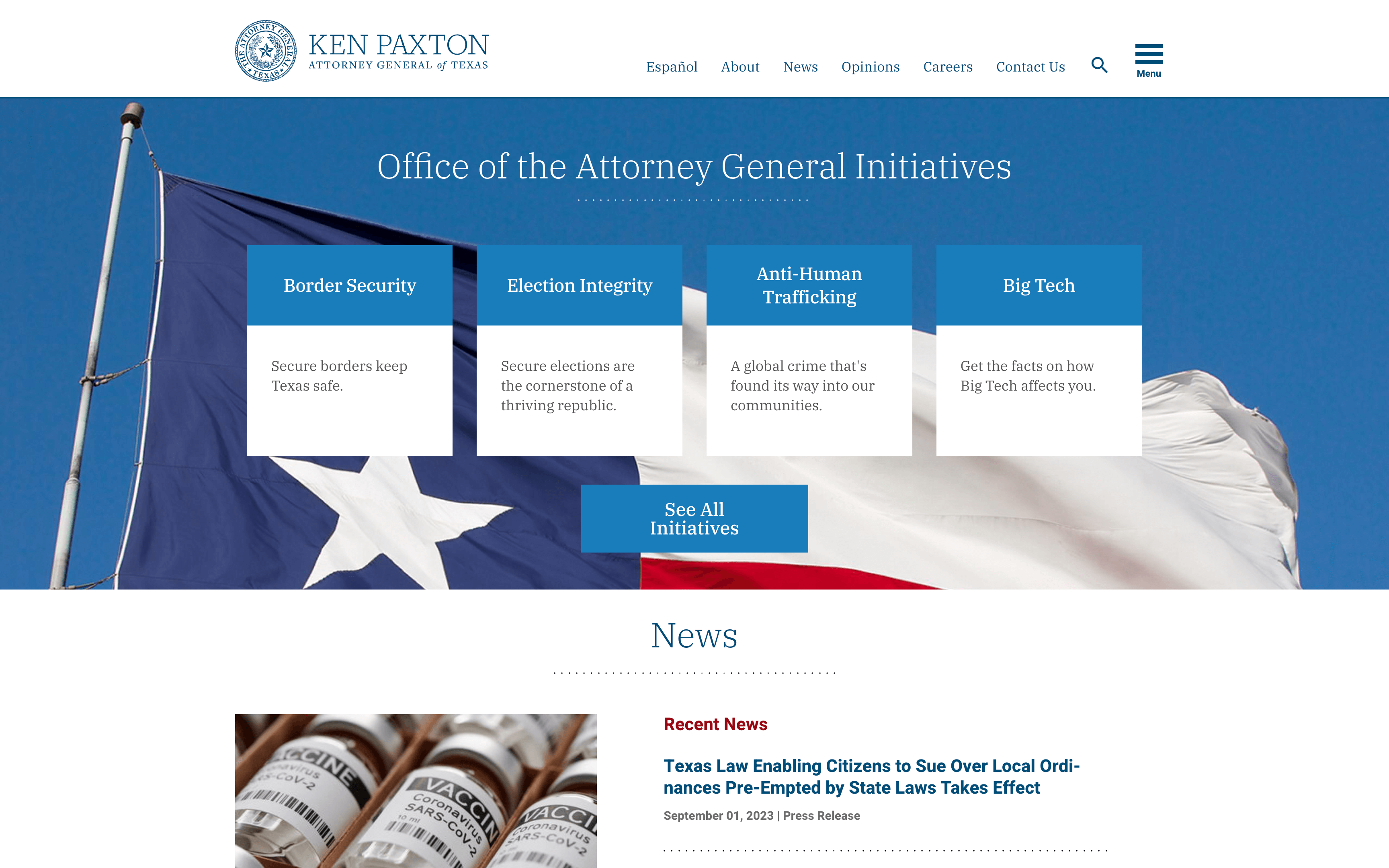The website screen showcases the homepage of Ken Paxton, Attorney General of Texas. In the top left corner, the logo is displayed adjacent to the name "Ken Paxton" in bold lettering. To the right, a navigation bar features links for "About," "News," "Opinions," "Careers," and "Contact Us," along with a language selection option, a search icon, and a pull-down menu.

Dominating the main splash screen is an image of a billowing American flag set against a clear blue sky. Superimposed over this backdrop is the text "Office of the Attorney General Initiatives" in white lettering. Below this header, a grid of squares presents various key initiatives: the first square on the left is labeled "Border Security," the second "Election Integrity," the third "Anti-Human Trafficking," and the fourth "Big Tech." The upper portions of these squares are blue, mirroring the sky but in a slightly lighter hue, while the lower portions are white.

Beneath these initiative squares is a blue rectangle with small white text that reads, "See All Initiatives." Further down, the webpage transitions to a white section centered around the heading "News." To the left under this heading is an image of various vaccines labeled with terms such as "Coronavirus," "SARS," and "COVID-2." Adjacent to the image is a recent news headline: "Texas law enabling citizens to sue for local ordinances pre-empted by state laws takes effect."